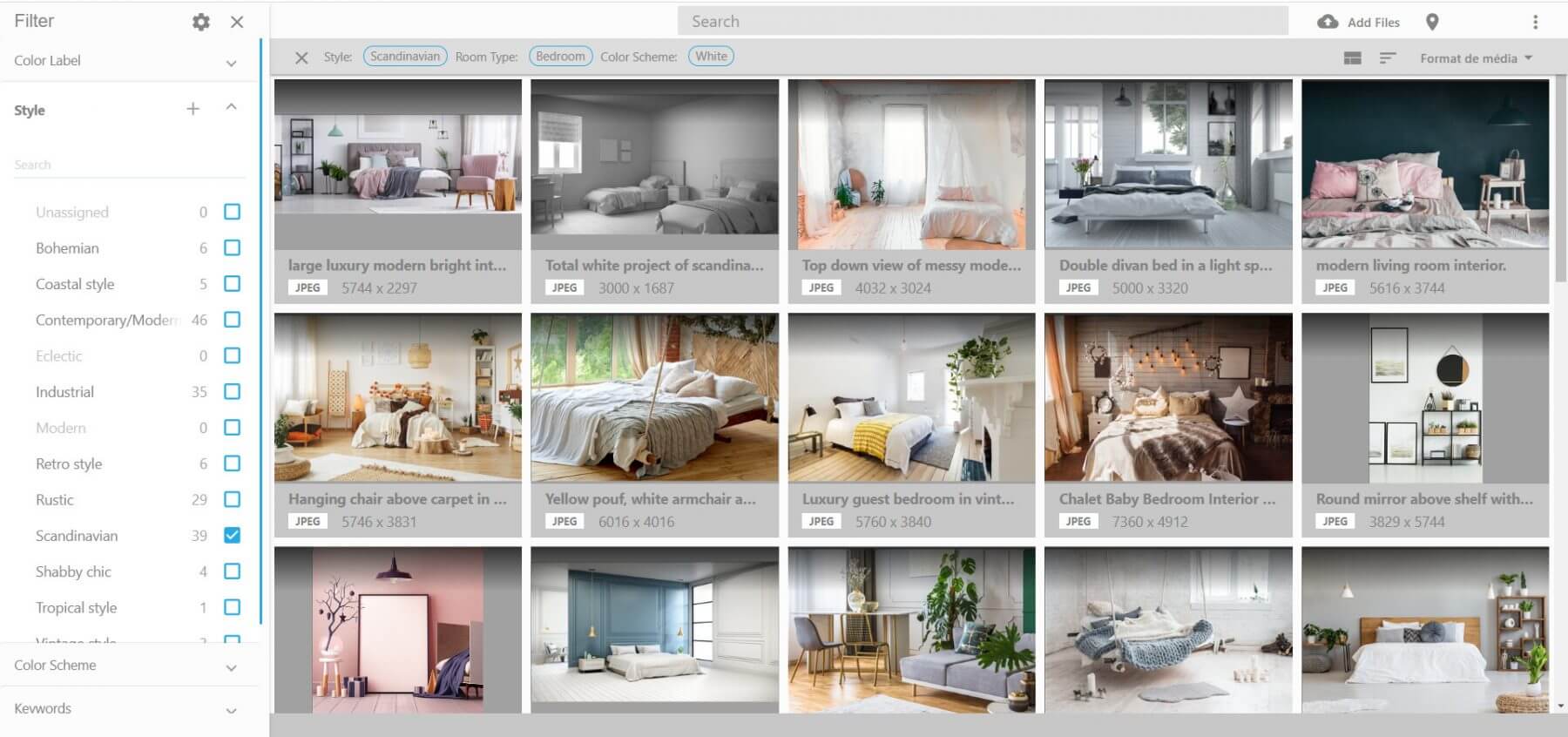This screenshot captures a detailed segment of a web browser dedicated to interior design, specifically focusing on bedroom aesthetics. The interface is divided into two main sections. On the left, the filter panel allows users to refine their search based on color and style categories. The filter section begins with a search bar for entering a preferred style, followed by a comprehensive list of various design styles. Each style entry features a small blue-outlined checkbox and an accompanying number indicating how many examples are available. 

At the top of the list, the "Unassigned" category is grayed out and shows zero entries. Following it, "Bohemian" has six entries available, indicated with a blue-outlined box next to the number. Other notable styles include "Coastal," "Contemporary," "Modern" (with zero entries), "Eclectic" (grayed out), "Industrial" (showing 35 entries), and "Retro" (showing six entries).

On the right side, occupying the larger portion of the browser, there are three rows displaying a total of 15 bedroom images, each portraying diverse design aesthetics. Every image includes a brief description and the specific dimensions, such as "2000 x 367," allowing viewers to gain both visual inspiration and practical information for their interior design projects. This user-friendly web page serves as a comprehensive resource for anyone interested in exploring and selecting bedroom design styles.